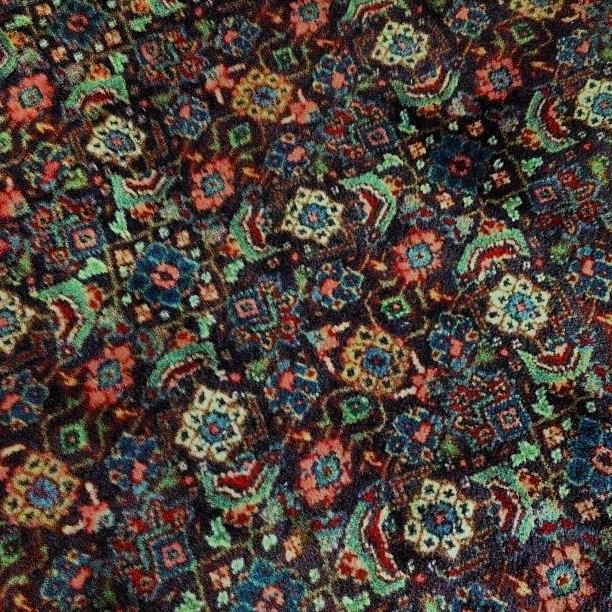This is a close-up color photograph of a richly patterned, potentially hand-woven, vintage-style rug taken from above. The intricate design features a black background, decorating the rug with squares, diamonds, rectangles, and various flower-like shapes and petals. The rug showcases a woven pattern that's continuous across all four sides of the image, dominated by hues such as blue, red, pink, green, white, orange, mint green, dark brown, and yellow, although the colors appear somewhat faded. Notably, decorative elements include rows of white circles juxtaposed with diamond shapes, as well as blue petals encircling pink centers. Some diamonds feature smaller diamonds within, adding to the elaborate complexity. Conversely, two of the rug's corners are notably dirty, highlighting signs of wear on the otherwise ornate piece.